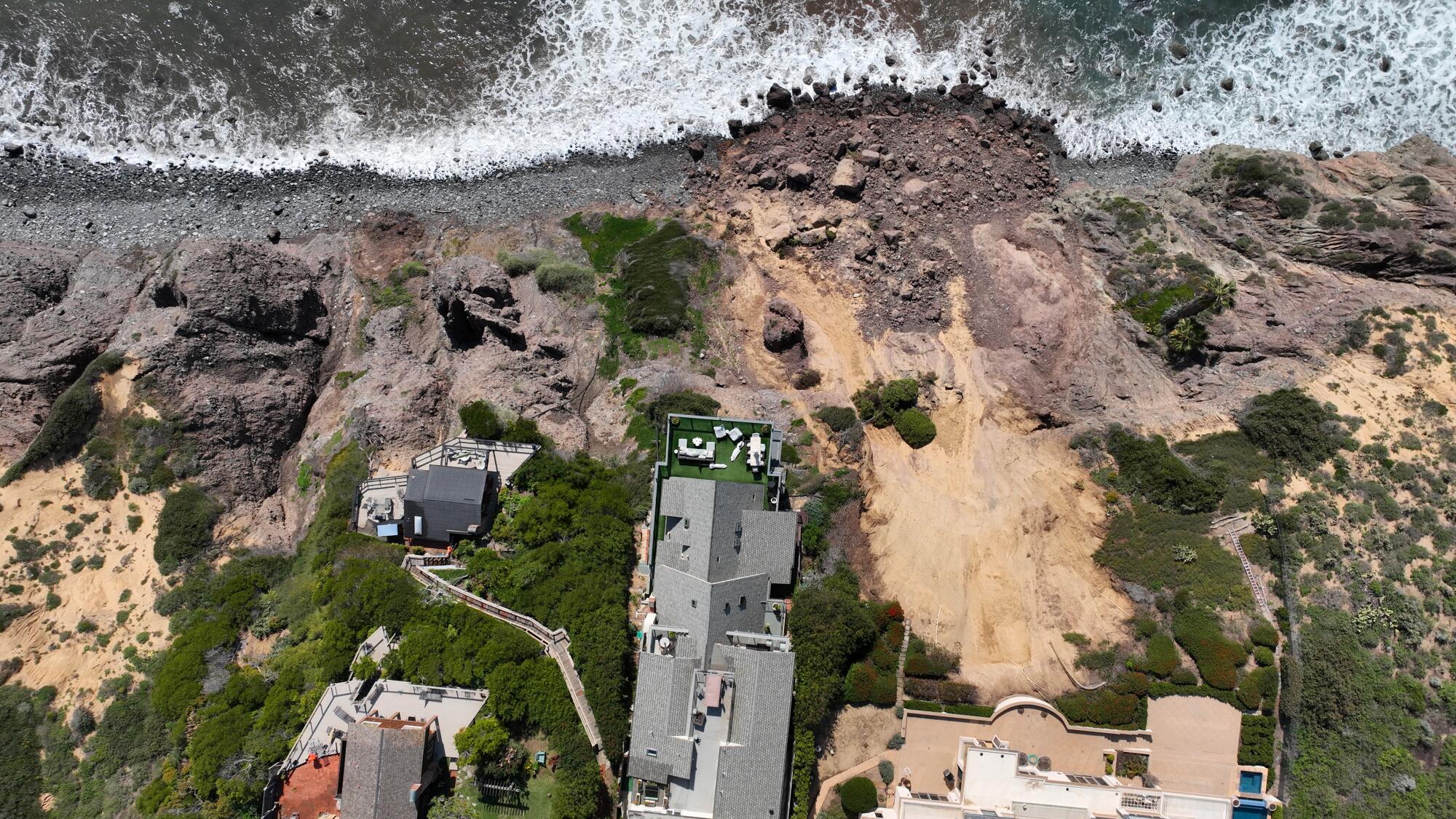This aerial shot captures a dramatic coastal scene featuring a row of houses perched precariously on a hilltop above a rugged cliff that descends sharply into the ocean. The upper half of the image showcases the dark bluish-gray waters, their white foamy waves relentlessly crashing against the rocky shoreline below. The cliff's composition includes a mix of reddish-brown and gray rocks, indicative of a recent landslide where some rocks have tumbled down. Atop the hill, a series of houses stand prominent – most notably a long, thin house with a gray roof positioned vertically towards the water's edge. This house appears dangerously close to the precipice and the potential landslide area. Nearby, a large tan section of another home is partially visible to the right, while further left are darker-colored homes, somewhat obscured. Patches of greenery, including trees, bushes, and other vegetation, dot the landscape around the homes, contrasting with the dirt and rocky terrain. The overall lighting is bright, suggesting a sunny day.